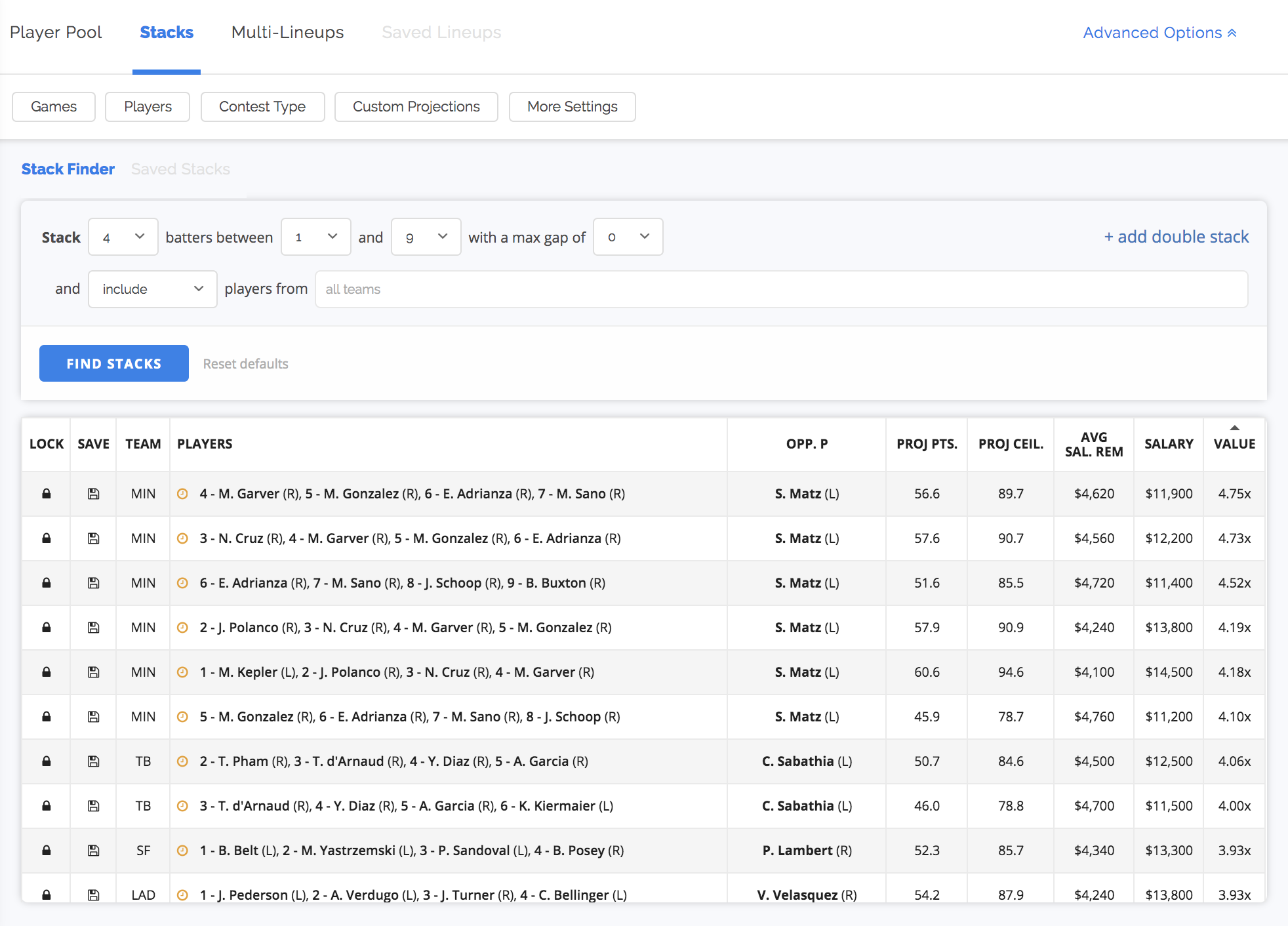**Caption:**

The interface appears to be a betting or gaming platform focused on team and player statistics. The top left section likely involves betting on teams. The main screen displays several sections, with the top including tabs for "Teams," "Pool Player," "Stacks," "Multi Lineups," and "Saved Lineups" to the right. An "Advanced Options" tab is also present on the same row.

Below the blue-highlighted "Stacks" tab, the rest of the options ("Multi Lineups," "Saved Lineups," etc.) are grayed out against a predominantly white background. Further down, a secondary navigation menu lists "Games," "Players," "Contest Types," "Custom Projections," and "More Settings."

The "Stack Builder" section below includes various configurable options:
- **Stack Finder:** Allows setting parameters like the number of players in a stack, denoted with pull-down menus between 1 and 9 and a maximum gap setting.
- **Include Players From:** A pull-down menu where you can select specific teams.

On the right, there is a link labeled "+ Add Double Stacks" in blue. Below that, a blue button labeled "Find Stacks Result Defaults" is evident.

Additional elements at the bottom include:
- **Lock Save Team Players**
- **OPP (Opponent)**
- **PP (Projected Points)**
- **Average Salary (Sal)**
  
These elements facilitate building and managing fantasy sports lineups or betting strategies.